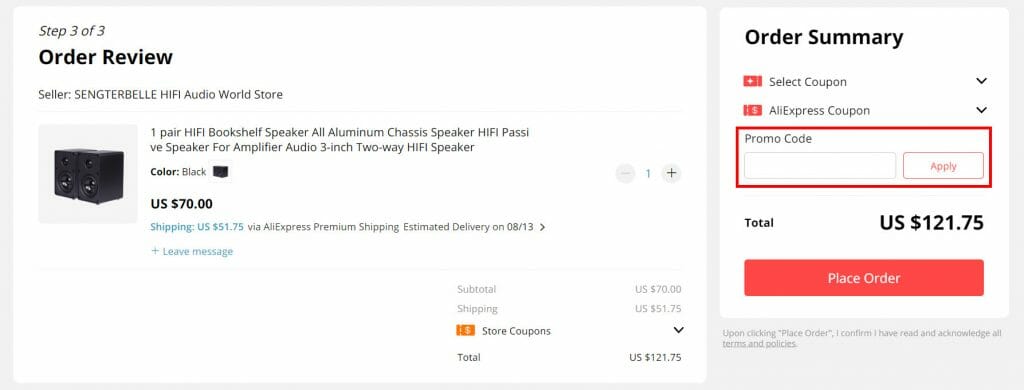**Order Summary: Step 3 of 3 - Review Order**

**Seller:** SingTribble, Hi-Fi Audio World Store

**Item Purchased:** 
- **Product:** One pair of Hi-Fi Bookshelf Speakers
- **Description:** All aluminum chassis, Hi-Fi passive speakers designed for use with an amplifier, featuring a 3-inch two-way Hi-Fi audio configuration

**Cost Breakdown:**
- **Item Price:** $70.00
- **Shipping Cost:** $51.75 (via AliExpress)
- **Total Cost:** $121.75

**Note:** The total cost appears to include a disproportionately high shipping fee, amounting to nearly as much as the speakers themselves. Despite this, the purchase has not yet been finalized, as indicated by the "Place Order" button at the bottom of the summary.